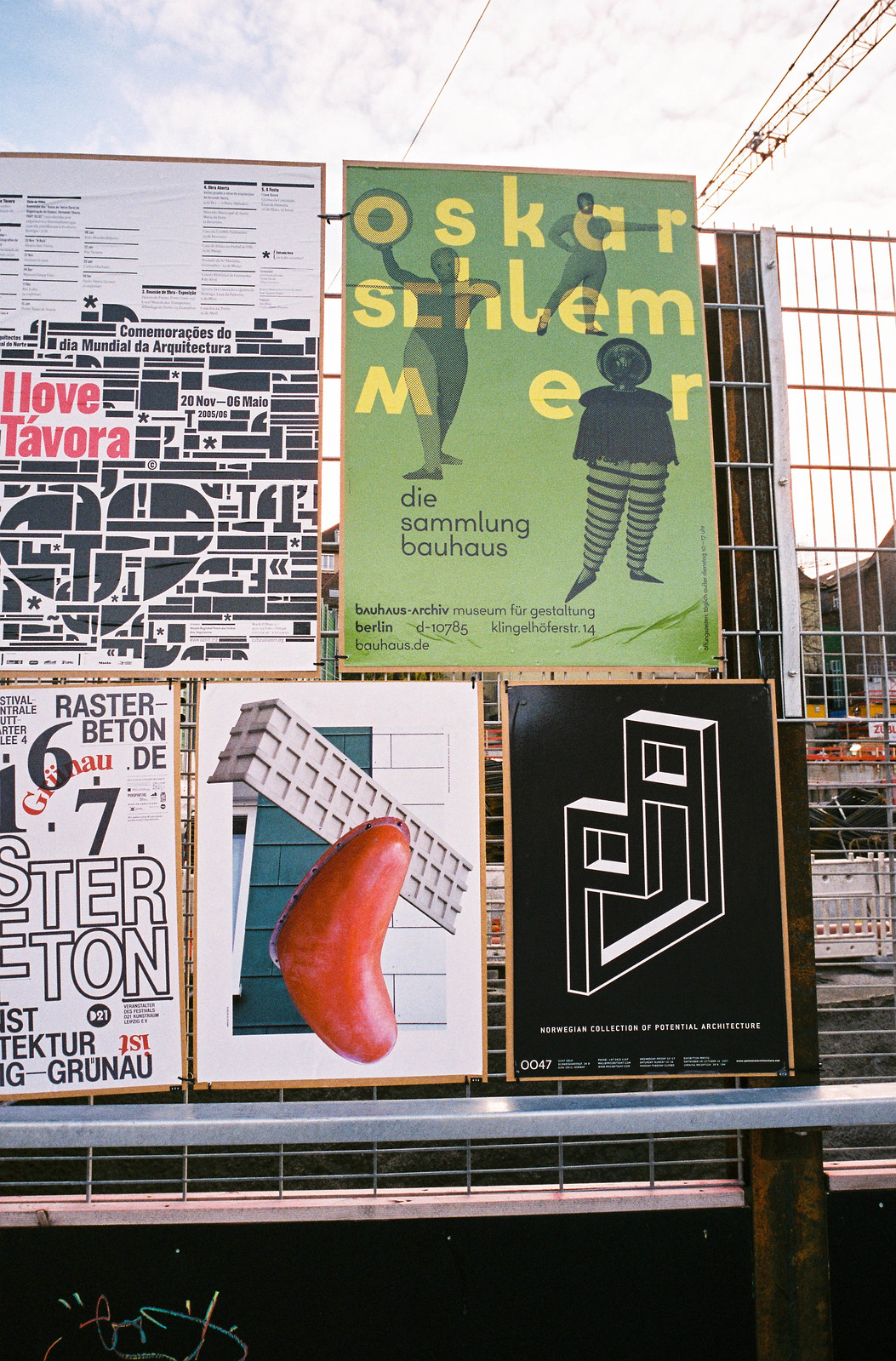This detailed daytime outdoor photograph captures a series of five eclectic posters affixed to a wire fence that resembles industrial barriers often used around construction sites. The sky, mostly overcast with a sliver of blue in the top left corner, sets a contrasting backdrop to the vivid content displayed on the posters.

Dominating the top right of the display is a light green poster adorned with yellow and black text, promoting Oscar Schillemeyer. This poster features three figures, possibly dancers. Adjacent to it on the left, a minimalist black and white design declares "I Love Tavora," with a bold black heart symbolizing the love for this unknown entity.

On the lower row, three posters stand out. To the left, a black-and-white abstract poster showcases geometric shapes with untranslated white text. Central to this lower trio is a poster with a white background, featuring a prominent red, bean-like shape and some green architectural elements that vaguely resemble shingles or doors. Finally, the bottom right poster displays geometric designs in black-and-white on a dark background, labeled in a foreign language—the text intriguingly mentions "the region collection of potential architecture."

Taken together, these posters create a tapestry of visual art and text against a functional wire fence, supported by a wooden pole and silver railing, with the overcast sky providing a muted yet complementary background.